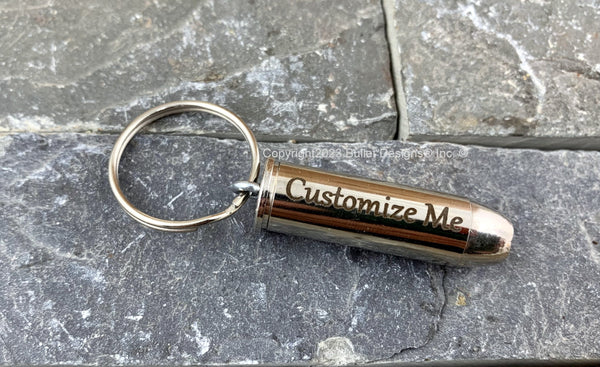The photograph captures a bronze-colored keychain resembling a bullet, lying on a gray stone surface composed of interconnecting paving stones. The metallic bullet keychain prominently features the engraved text "Customize Me" along its side. The keyring itself appears to be a brassy gold hue. The image includes an overlay watermark that reads, "Copyright 2023, Bullet Designs Incorporated," in faded white text. The setting and the clarity of the photograph suggest it could be used for listings on websites like Etsy.